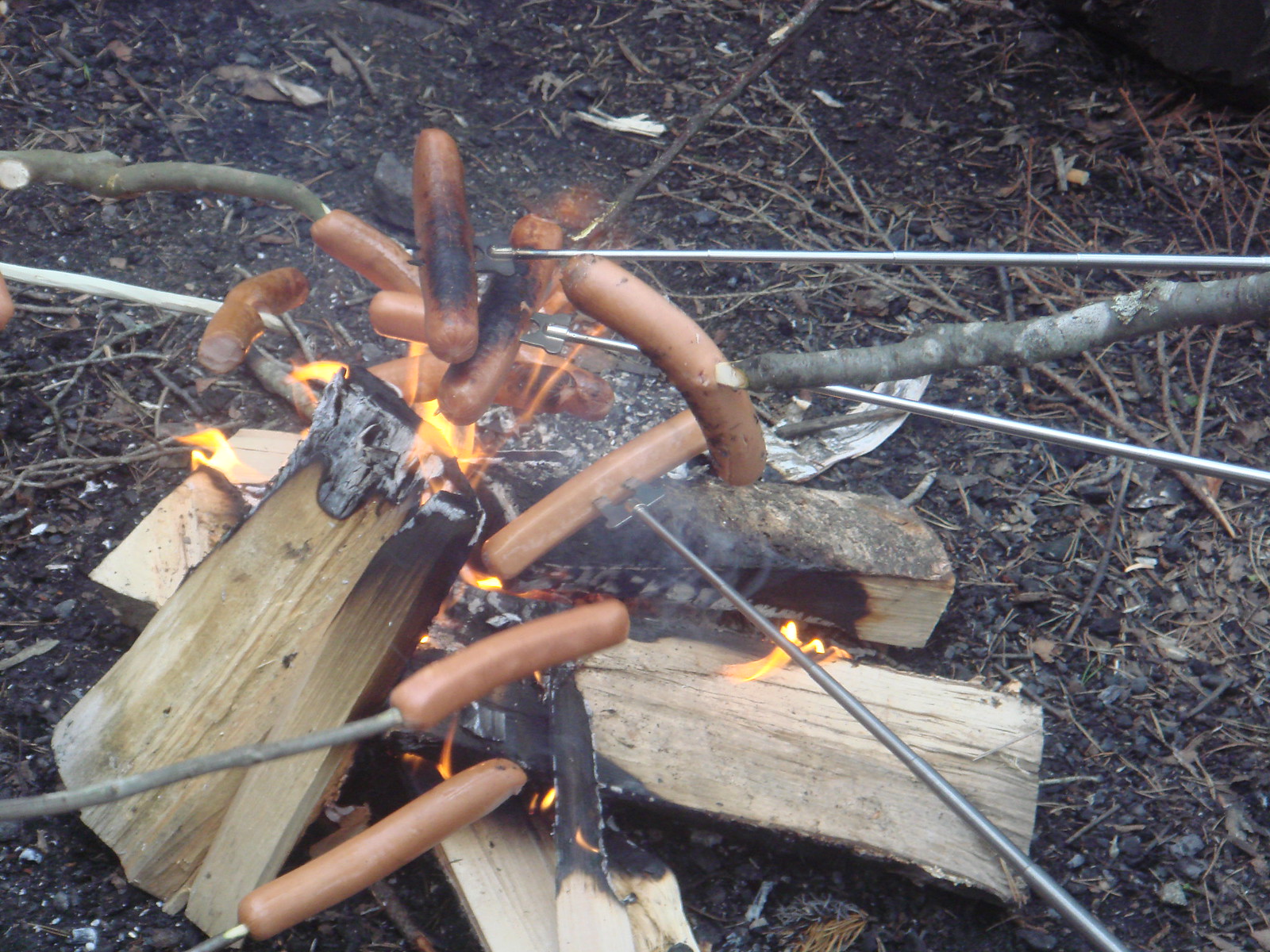This color photograph captures an outdoor scene during daylight, showcasing a rustic campfire on dark, mulch-like ground, scattered with dried pine needles, thin twigs, and white ash specks. The campfire consists of large split logs arranged in a triangular or teepee shape with low flames in the center. Several sticks and metal rods, both rough branches and silver metals, extend from the edges of the frame toward the fire. On the ends of these sticks are approximately ten hot dogs, some charred and browned, while others remain uncooked, indicating they were placed at different times. The ground around the fire is a mix of dark dirt, browns, and blacks, emphasizing the raw outdoor setting of this campfire cooking scene.